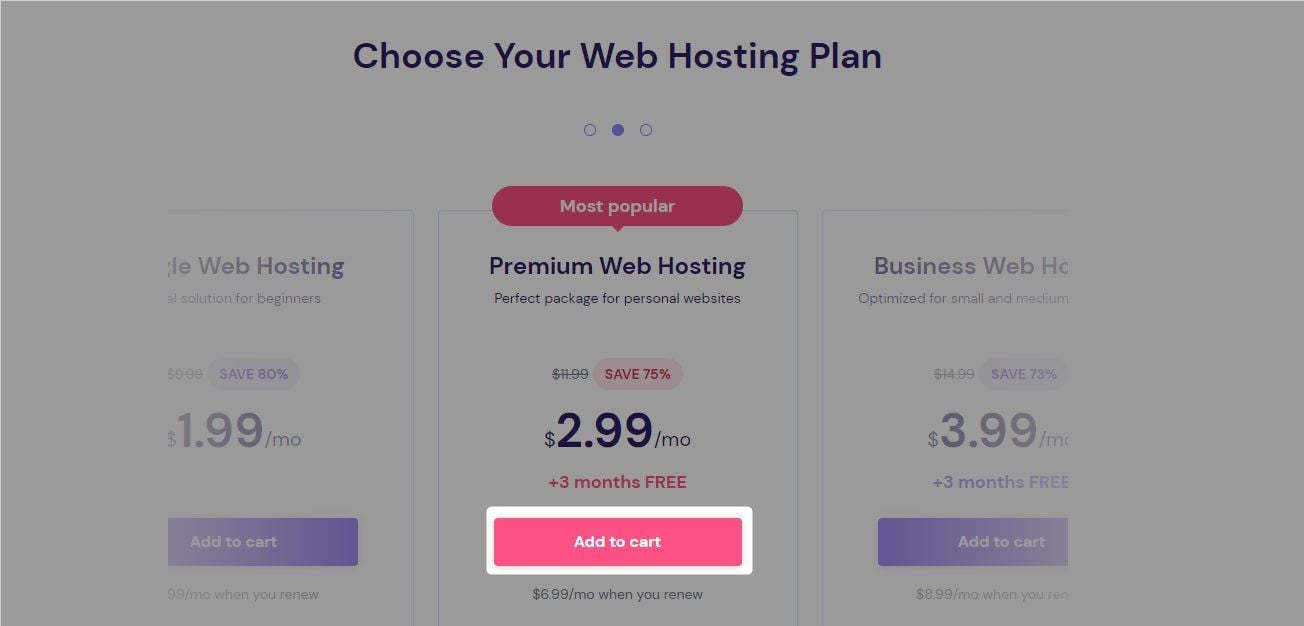The image is a screenshot of a computer screen displaying various web hosting plans. The background is predominantly grey and muted. Along the top, the text “Choose Your Web Hosting Plan” is prominently displayed in black lettering. Below this heading are three circles, where the central circle is solid blue, contrasting with the other two which are hollow and outlined in blue.

The middle section, accentuated as the focal point of the image, features a red elongated oval with the text “Most Popular.” This section, labeled "Premium Web Hosting," is described as the "Perfect package for personal websites." Originally priced at $11.99, this plan offers a 75% discount, bringing the cost down to $2.99 per month, along with an additional three months free, highlighted in red. A prominent red button below this displays “Add to Cart,” followed by a note that the renewal price is $6.99 per month, in black text.

On the left side of the middle section, there is a plan described as a solution for beginners labeled "Web Hosting.” It offers an 80% discount, making it $1.99 per month, with a renewal price undisclosed in the muted text.

On the right side, there is another plan suited for small and medium businesses labeled "Business Web." Originally priced at $14.99, it offers a 73% discount, reducing the price to $3.99 per month with three months free. This plan also includes a red “Add to Cart” button, with a renewal price listed as $8.99 per month in black text.

The central column is clearly the most emphasized, with bold, bright colors drawing attention away from the more subdued and less highlighted plans on either side.